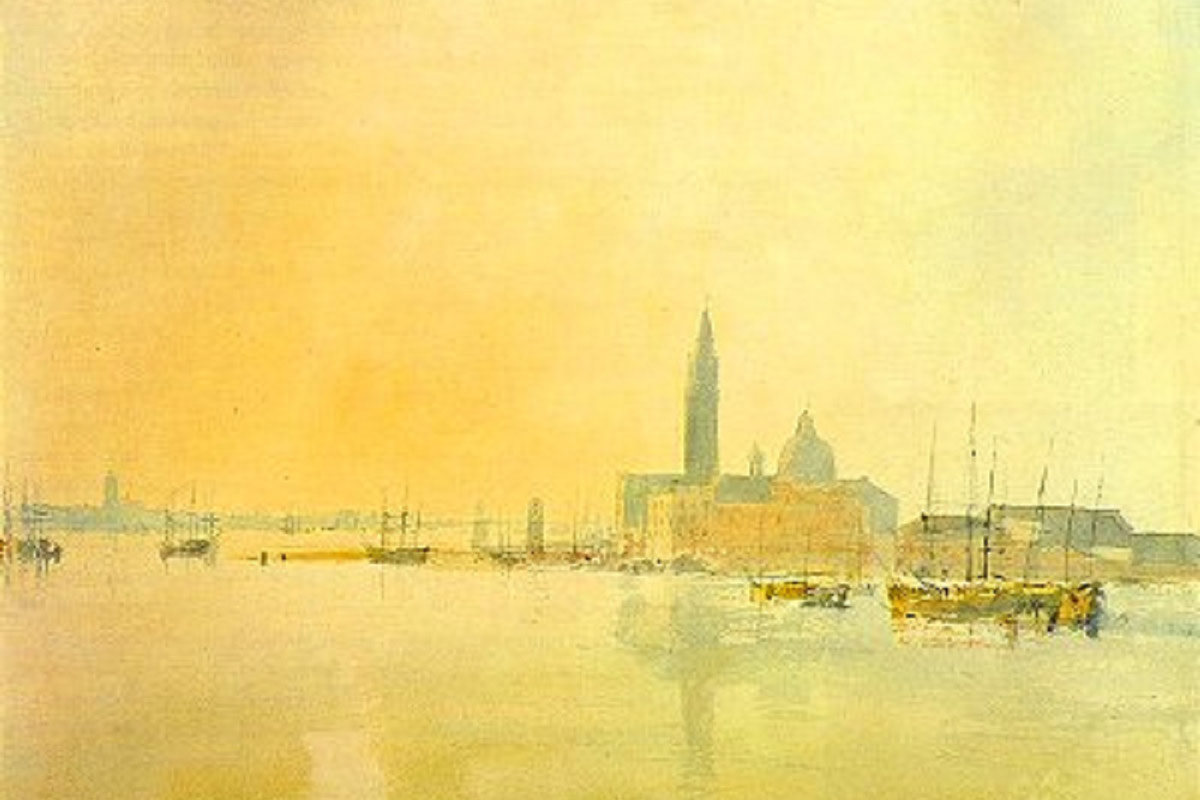This impressionistic watercolor painting depicts a coastal cityscape bathed in hues of yellow and orange, with traces of green. The sky and water seamlessly blend together in shades of pinkish-orange and yellow, creating a surreal, dreamlike atmosphere without clearly defined features. In the foreground, poorly defined boats with masts float on the orange-pink water. The city's skyline includes several buildings, with one prominent structure characterized by a tall, thin spire resembling a sword on top of a flat roof. This particular building, painted in green, contrasts with the adjacent orange building. Dark gray and shadowy black buildings can be seen towards the horizon, adding depth to the composition. The overall effect is a vivid, yet hazy portrayal of the city, where colors and forms merge together in an ethereal landscape.